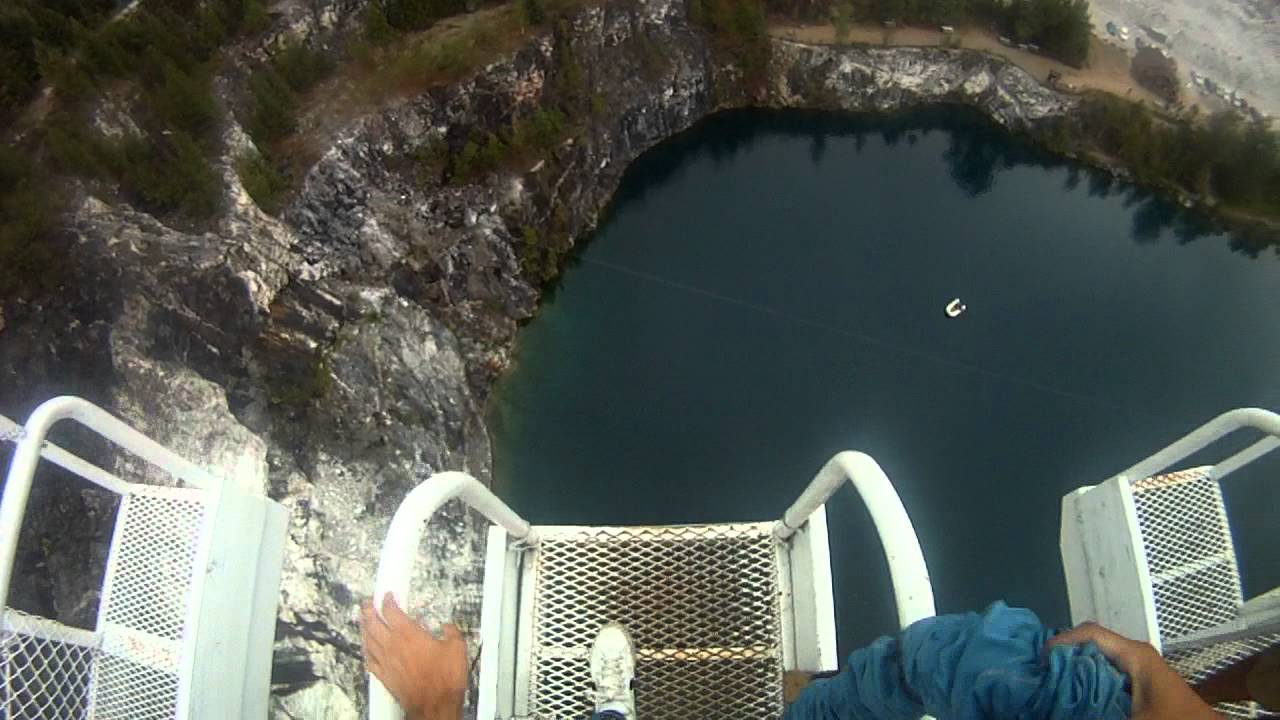The photo captures a scenic, high-angle view of a lake nestled in a rugged canyon landscape, framed by imposing cliffs and lush vegetation. Dominating the scene, the lake lies slightly off-center to the right, reflecting the tranquility of its surroundings. In the top right corner, a faint stretch of what appears to be a beach is just visible. The lower half of the photo features three white platforms constructed from corrugated metal, complete with mesh and handrails. Suspended precariously over the cliffs, these platforms suggest an extreme activity such as bungee jumping. Indeed, barely within the shot, the hands and feet of a man imply a daring jump is imminent, though no faces are visible. Additional elements include a white boat floating in the lake, possibly for safety or observation, and a mix of grayish-white rock formations and trees that embrace the water body around its perimeter.